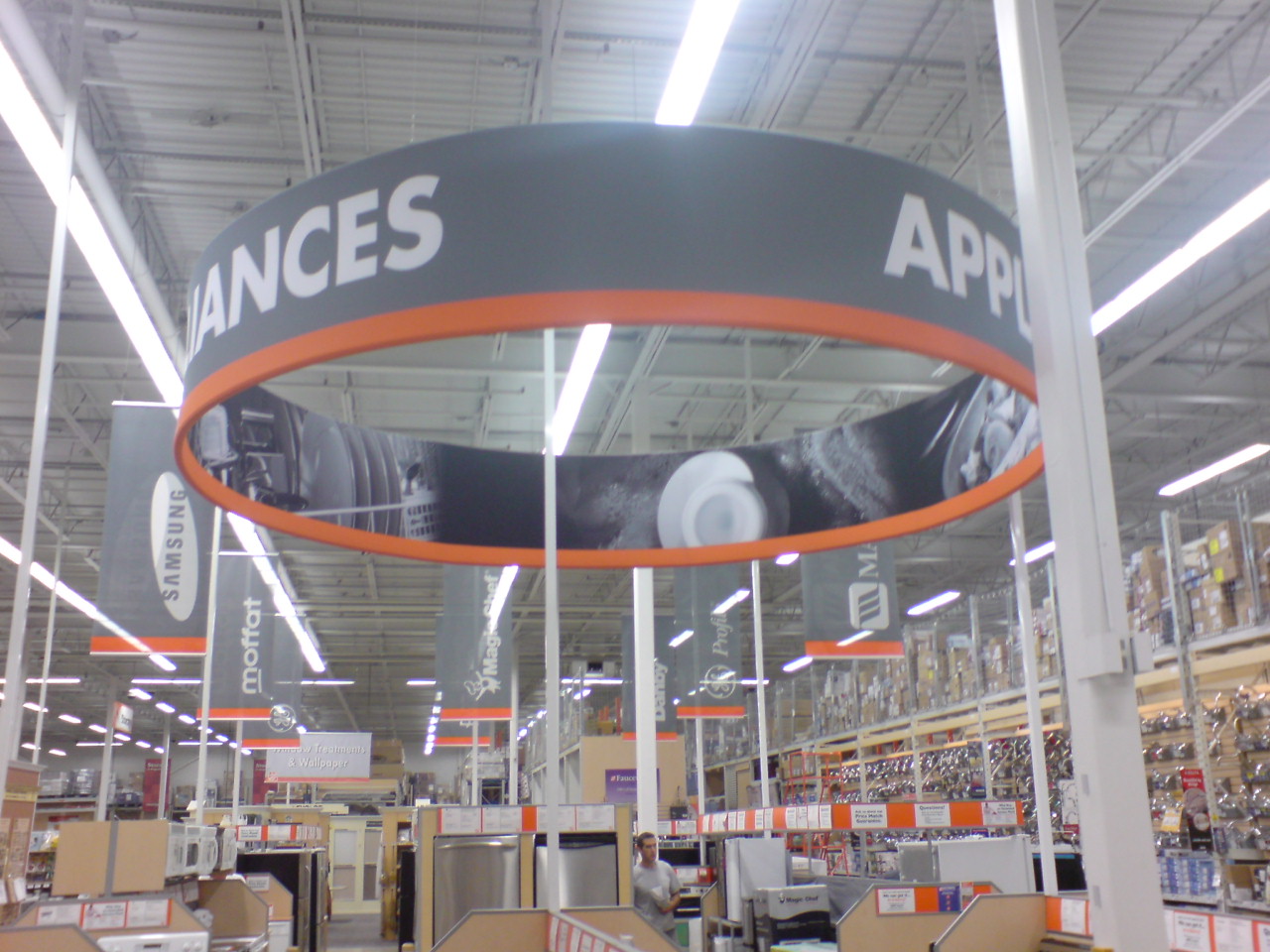This photo depicts the interior of what appears to be a Home Depot, distinguished by its characteristic tall ceilings with exposed metal rafters and long fluorescent lights. The recognizable orange and gray color scheme is predominant, along with large, hanging signs that display various brand logos such as Maytag, GE, Samsung, and Motorola. Central to the image is the appliance section, as indicated by a prominent circular sign with an orange border that reads "APPLIANCES." Below, an array of stainless steel refrigerators, white washers, dishwashers, and microwaves are neatly arranged. In the background, there are aisle signs for window treatments and wallpaper, reinforcing the impression of a hardware store. A man in a gray shirt, holding a book in his left hand, is seen walking through the appliance aisle, possibly inspecting the available products. The overall ambiance, with its red and white elements, further suggests a Home Depot environment.